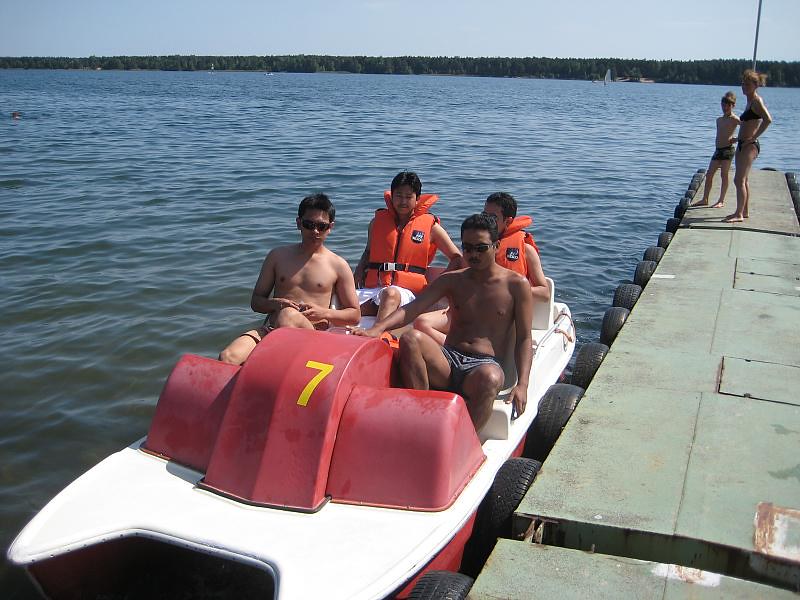In the color photo, a tranquil scene unfolds over a large, blue, ripply lake, with a thin border of light blue sky meeting the opposite shore lined with a stretch of trees from left to right. In the far distance, sailboats are faintly visible. 

Closer to the forefront, a floating dock with vertically lashed car tires acting as bumpers extends into the water. Standing on the grayish-brown dock are a woman in a bikini with her hair in a ponytail and her young son, both looking out at the lake. 

Moored beside the dock is a small paddle boat, which appears to be a rental. The boat is white with red trim and features a yellow number 7 on what seems like a car engine cowl, hinting at an engine disguised to house pedal mechanisms. In the boat's front, two shirtless men in swim trunks and sunglasses have their feet positioned in the pedal area, suggesting they will propel the boat. Two younger individuals wearing orange life vests occupy the rear seats. 

The serene blue water and sky create a peaceful backdrop for this leisurely lakeside moment.